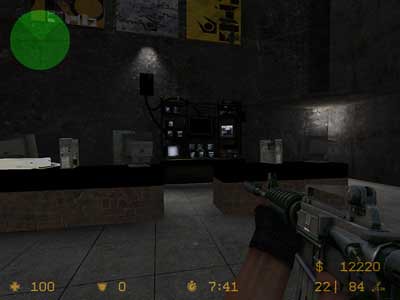Inside a store during nighttime, the environment is dim with subdued lighting. The floor is covered with large slate tiles, each approximately two and a half feet square. Several counters, some of which are backlit, line the space, contributing to an ambiance reminiscent of a jewelry store. However, the specific nature of the store remains ambiguous. Suspended from the ceiling are various banners or posters, the details of which are unclear. One poster on the right stands out with a yellow background. The store appears closed, with no active business taking place. The bottom of the image features numbers, and a green dot is visible at the top. There is a numerical detail "741" and what seems to be a date "12-2-20" possibly indicating when the photo was taken.